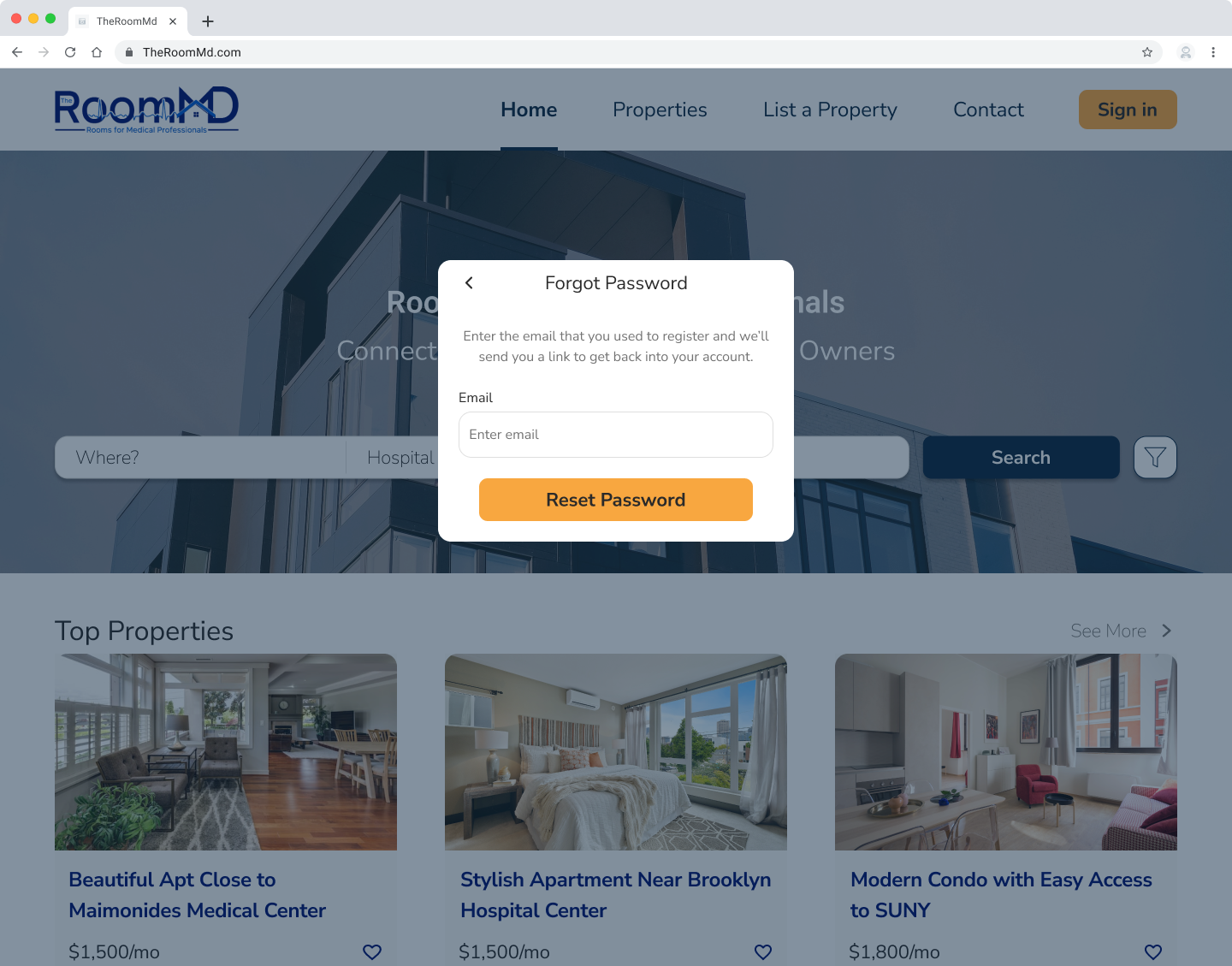The image showcases the homepage of RoomMD, a real estate website. The logo features the word "RoomMD" with the middle of the "M" designed to look like a house. The main navigation menu includes options such as "Home" (underlined in blue), "Projects," "List of Property," and "Contact." On the right side, there's an orange rectangle button with "Sign In" written in black. 

Below this, a white box prompts users with "Forgot password? Enter the email that you use to register and we'll send you a link to get back into your account." Below this prompt, there is an "Email" field followed by an orange "Reset Password" button.

The homepage also highlights top properties with three pictures of apartments. The listings include:
1. A beautiful apartment (APT) close to Maimonides Medical Center, available for $1,500/month.
2. A stylish apartment near Brooklyn Hospital Center, available for $1,500/month.
3. A modern condo with easy access to SUNY (State University of New York), available for $1,800/month.